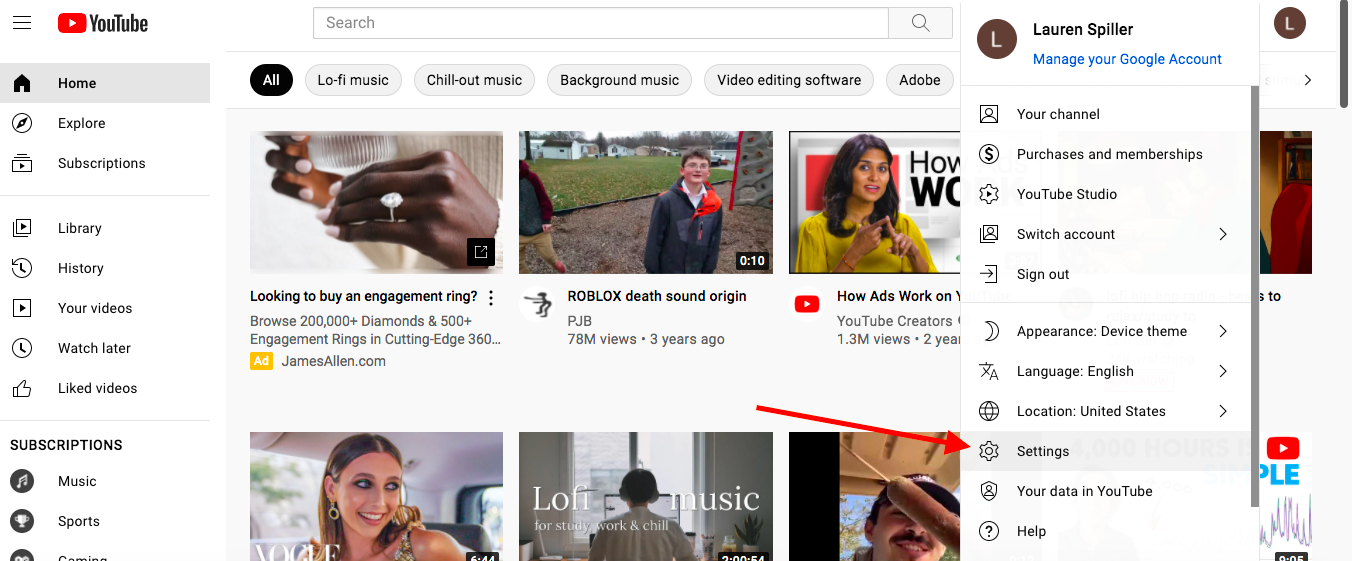Here is a detailed and cleaned-up description of the image of the YouTube website:

In this image of the web-based version of the YouTube site, we see a clean white background. In the top left corner, there is a "list" button next to the YouTube icon and symbol. The top right corner shows the profile tab, which has been clicked, revealing the user's name, Lauren Spiller. This drop-down menu includes options such as "Your channel," "Purchases and memberships," "YouTube Studio," "Switch account," "Sign out," "Appearance: Device theme," "Language: English," "Location: United States," "Settings," "Your data in YouTube," and "Help."

The center of the image features thumbnails of various videos. At the very top, there are tabs labeled "All," "Lo-fi music," "Chill out music," "Background music," "Video editing software," and "Adobe." The search bar, located in the top center, is currently blank. 

On the left-hand side of the screen, there are several navigation tabs, including "Home," "Explore," "Subscriptions," "Library," "History," "Your videos," "Watch later," and "Liked videos."